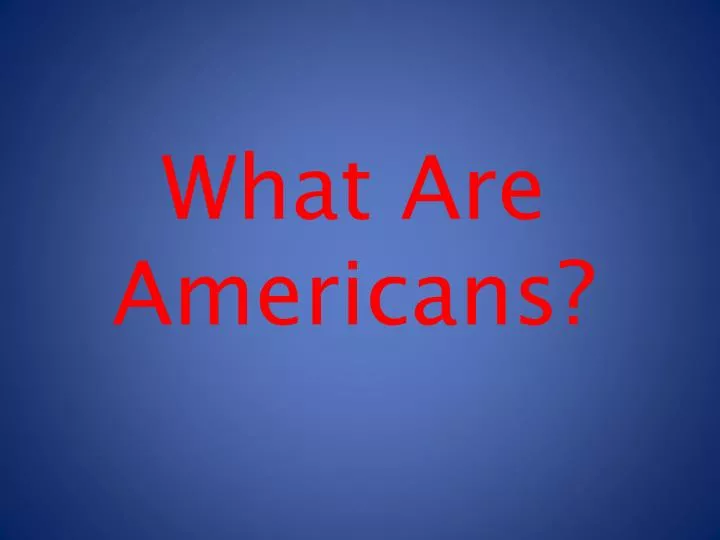The image displays a single slide that appears to be from a PowerPoint presentation. The background features a deep blue gradient, starting darker at the edges and gradually becoming lighter towards the center where the text is located, with a distinctive vignetting effect in the corners. In the middle of the slide, written in large, medium-thickness red font, is a provocative question presented over two lines. The text reads: "What are Americans?" with each of the first letters—W, A, and A—capitalized, while the rest of the letters are in lowercase. The overall layout and style suggest it is intended to spark philosophical discussion or debate, potentially aiming to evoke various perspectives on American identity, possibly from those outside the United States.